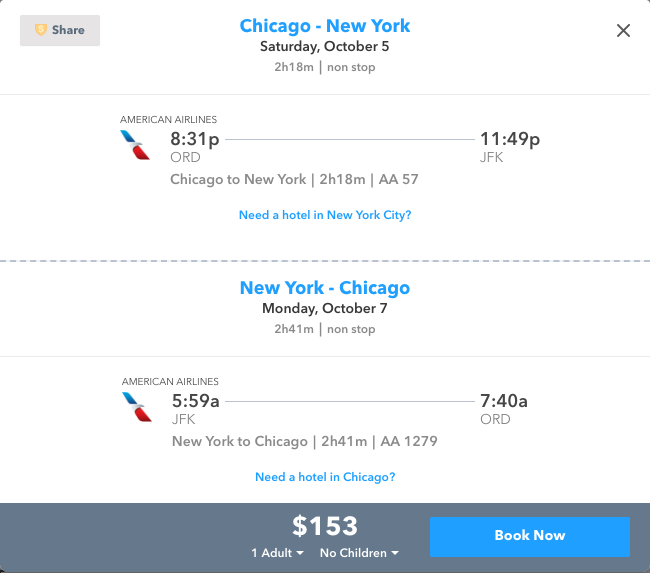Detailed Caption:

The image displays a flight schedule webpage by American Airlines, showcasing travel details for a round trip between Chicago and New York. At the top, the webpage header is prominently marked in blue with the text "Chicago to New York." Just below, the date is specified as Saturday, October 5th, with the flight duration noted as 2 hours and 18 minutes for a non-stop trip. On the left side of the header, there is a share button, and an "X" icon is visible on the right side.

In the middle section, the airline's name, "American Airlines," is displayed, along with specific flight details: departing from Chicago O'Hare International Airport (ORD) at 8:31 p.m. and arriving at John F. Kennedy International Airport (JFK) in New York at 11:49 p.m. The flight number is indicated as AA57. Beneath this information, a clickable blue link suggests, "Need a hotel in New York City."

Further down, the return flight is outlined, slated for Monday, October 7th. The return trip is a 2 hours and 41 minutes non-stop journey. It mentions an American Airlines flight departing from JFK at 5:59 a.m. and arriving at ORD at 7:40 a.m., with the flight number AA1279. Another blue clickable link asks, "Need a hotel in Chicago?"

Towards the bottom of the page, a gray box highlights the fare information: $153 for one adult without children. Next to this, options to adjust the number of travelers are provided. To the right, a blue button labeled "Book Now" is centrally positioned, indicating it can be clicked to proceed with the booking.